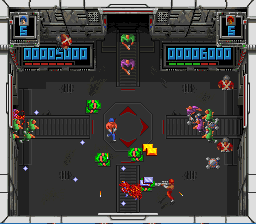This image is a detailed screenshot from a highly pixelated, top-down video game. The background is predominantly black with a textured gray wall at the top, which features a central opening where several characters are emerging—two in green shirts and two in purple shirts. In the middle of the scene, there's a square playing area with a black floor adorned with red features and lime green shapes marked with an orange stripe.

On the left and right sides of the image are rectangular scoreboards with block numbers in blue, displaying 0 0 0 0 5 0 0 0 on the left and 0 0 0 0 6 0 0 0 on the right. Both sides also have a blue "5" positioned above the scoreboards. At the center of these scoreboards are two shield-like icons, one green and pink and the other pink.

Amidst the gameplay area, several characters, each depicted as simple, tiny blocks in various colors, are visible. A player in red with a green and purple gun emitting fire stands out, alongside another character in orange and blue. Additionally, there are small red ovals with thick white Xs through them. The simple graphic style includes characters in red, slate gray, green, and pink, emphasizing the non-photorealistic nature of the game.

At the very top, likely the game's title and logo appear, rendered in turquoise blue, though the text is illegible. The overall scene captures a dynamic moment, illustrating the game's straightforward, pixelated artistry and chaotic, action-packed environment.